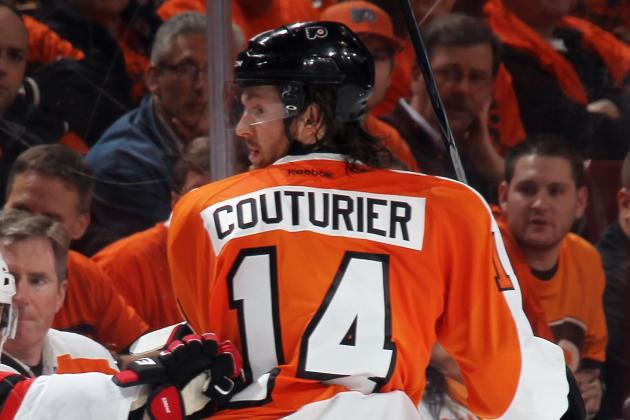The color photograph captures a Philadelphia Flyers hockey player, identified as Couturier with the name "COUTURIER" in capital black letters on a white name tag on his back. He is wearing an orange and white jersey with the number 14 in white with black borders. The player, who has long black hair, looks to his left, making his face partially visible. He sports a black helmet with a clear shield and the Flyers logo, and he holds a black hockey stick. Surrounding the rink, separated by glass, is a vibrant crowd, many clad in Flyers merchandise, with some wearing regular clothes. Notable is a man in a blue shirt with glasses and gray hair. Another hockey player appears to be grabbing onto Couturier. The scene emphasizes the intensity of the game and the audience's engagement.